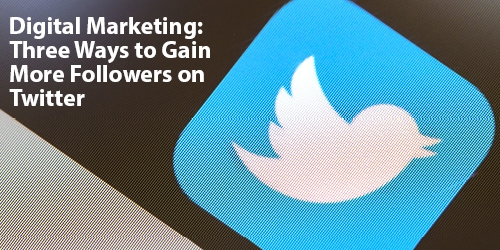This image is a screenshot of a Twitter advertisement. The background features a two-tone design with a predominant dark brownish color, transitioning to a grayish hue at the bottom left corner. At the top left-hand side of the image, there is a white text that reads "Digital Marketing;" followed by the lines "Three Ways to Gain," "More Followers on," and "Twitter." Positioned midway on the right-hand side of the screenshot is the iconic Twitter logo, which is displayed in light blue with a white, filled outline of a tweeting bird. Notably, the bird logo appears slightly off-centered and tilted to the right, giving the impression that it is facing downward. The image itself is rectangular in shape and not perfectly square, with a slight blur adding to the overall effect. This tilt and blur might be intentional, suggesting a dynamic and casual approach typical for social media advertisements.